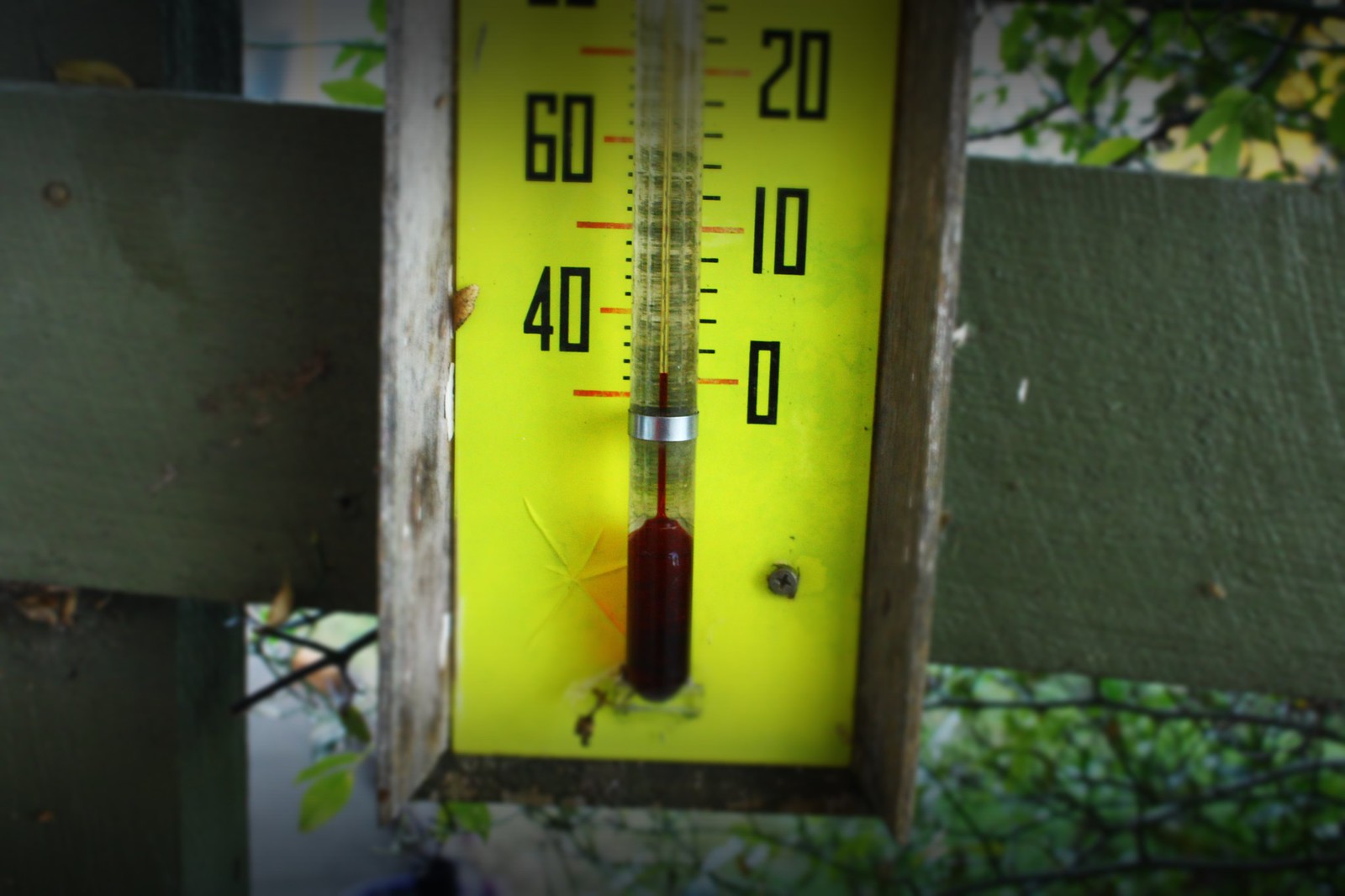This close-up image features the lower part of an outdoor thermometer mounted on a wooden surface, possibly a fence. The thermometer's background is a bright yellow, with black numerals indicating the temperature. Orange and black lines mark the temperature indicators, and the device is encased in a wooden-like frame. The red dye in the thermometer is clearly visible at the bottom, showing a temperature of around zero degrees. On the right-hand side, the visible numbers are 0, 10, and 20, while the left side shows 40 and 60, all in black. In the blurred background, you can faintly see trees and leaves, suggesting that the thermometer is located outdoors, likely in a residential area. However, the extreme close-up nature of the photo obscures the broader setting.